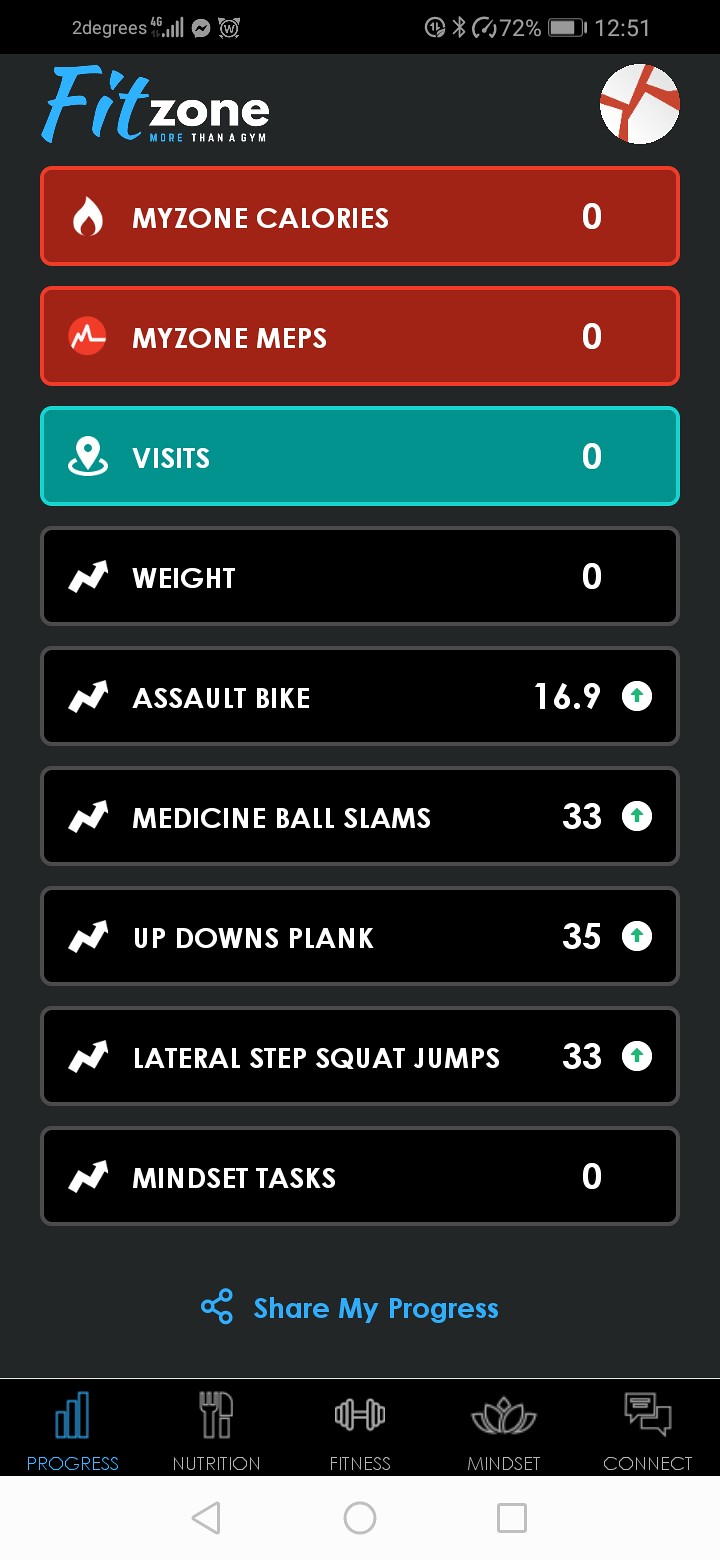The image is a screen capture of a mobile health and exercise app called FitZone, with the tagline "more than a gym" displayed prominently at the top. The background is a dark gray, giving the app a sleek and modern look. Across the top, in blue text, you see the word "fit," followed by "zone" in white, "more" in blue, and a gem icon in white.

The primary content consists of multiple rectangles with colored edges, each containing specific fitness data or sections. At the very top, two red rectangles list "My Zone Calories, Zero" and "My Zone M.E.P.S., Zero." Below these, a turquoise rectangle states "Visits, Zero." Further down, a black rectangle displays "Weight, Zero."

Continuing down the screen, there are several more rectangles covering various fitness activities: "Assault Bike," "Medicine Ball Slams," "Up Downs," "Plank," "Lateral Step," and "Squat Jumps." These entries are lined with icons representing each activity, such as an arrow, a direction symbol, a graph, a fire, weights, a plant, and fork and knife icons. The colors of these sections vary, with black, white, light blue, red, and light green making up the palette.

At the bottom of the screen, there is an option to "Share My Progress," indicating the app's social or community features. Various additional icons appear at the base of the screen, integrating overall navigation and additional resources related to mindset tasks, progress, nutrition, fitness, and connectivity. The entire layout seems to represent a home screen for a versatile and comprehensive fitness tracking application.